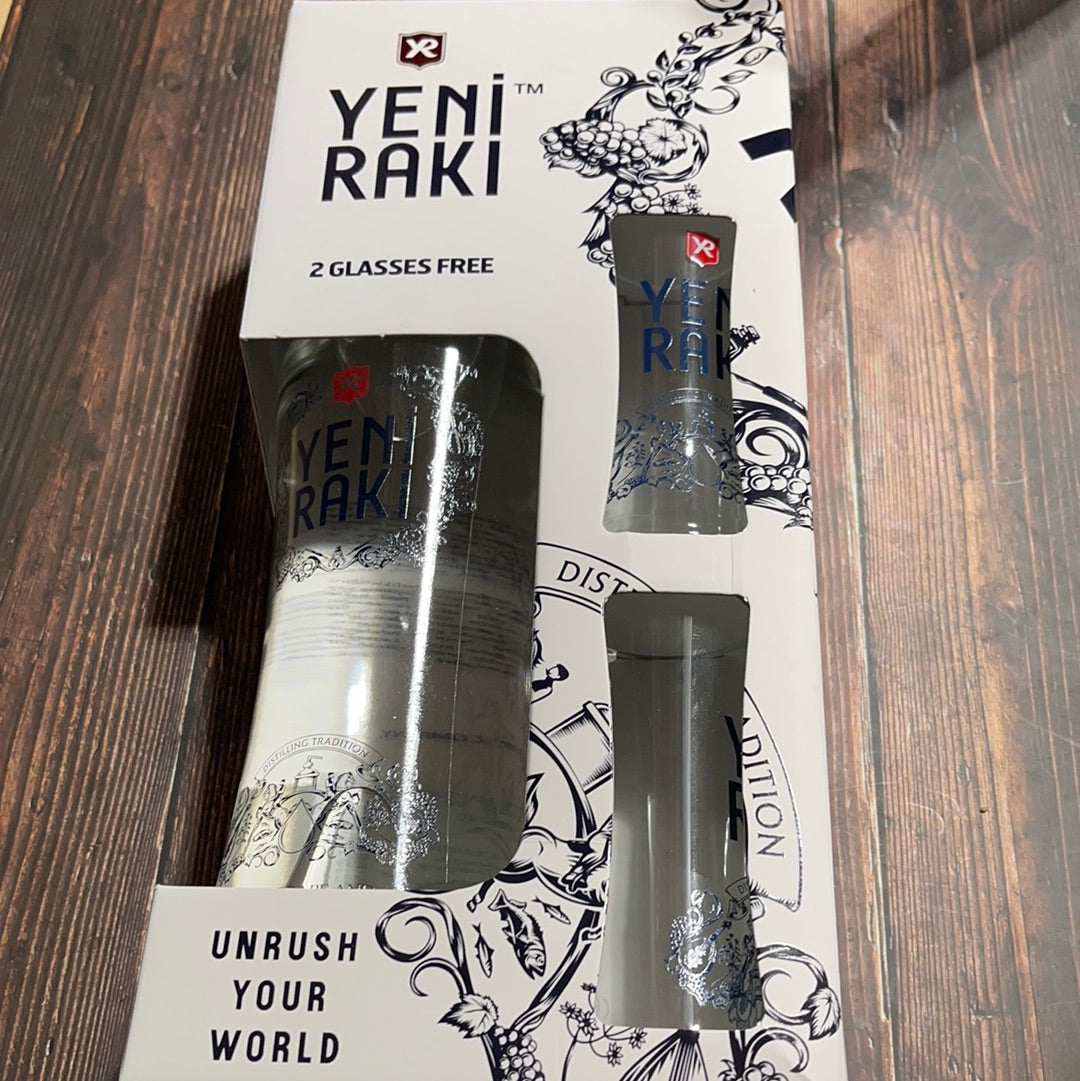The image depicts a cardboard box set with an off-white color, designed to attractively package a glass bottle and two shot glasses, both included with a promotion of "two glasses free." The box prominently features the brand name, Yeni Raki (spelled Y-E-N-I-R-A-K-I, with 'Yeni' on the first line and 'Raki' on the second), in condensed black text at the top left. Below this text, there's a cutaway viewport which reveals a tall, cylindrical glass bottle on the left. The bottle is adorned with a black logo that combines a stylistic Y and R in a coat of arms and is surrounded by intricate filigree decorations of vines and leaves. On the right side of the box, there are two additional vertical cutaways positioned on top of each other, each showcasing one of the included shot glasses, which also feature the same Yeni Raki branding and decorative filigree designs. At the very bottom of the box, both on the left-hand side and among the decorations, the text "Unrush Your World" is visible. The entire box set is placed on a wooden table, adding a rustic touch to the presentation.